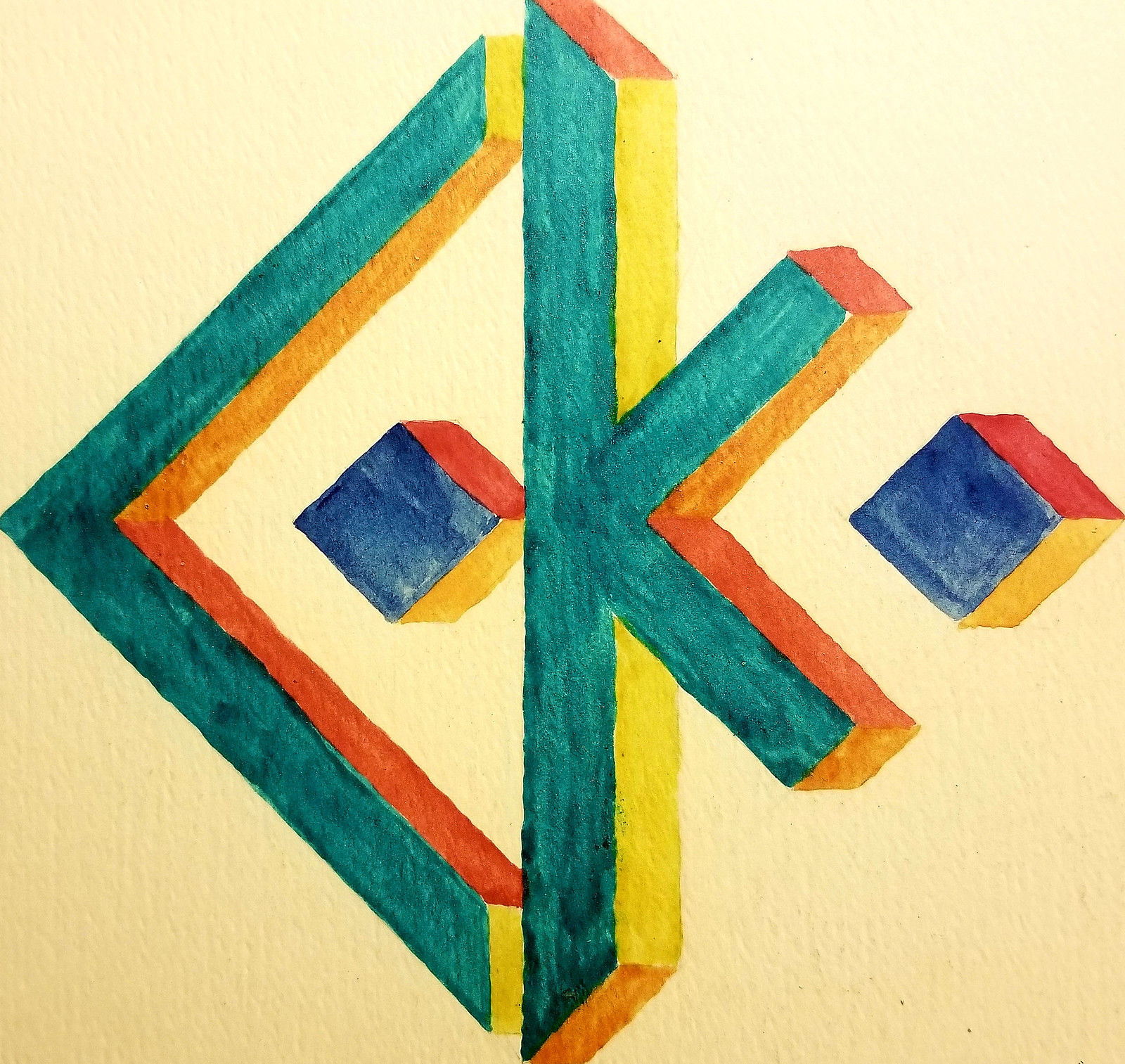This vibrant and abstract artwork features a colorful fish-like figure set against a light tan background. The body of the fish is composed of expressive shades of teal, orange, and yellow. Intriguingly, there is a cube embedded within the fish's body, displaying a spectrum of blue, orange, and yellow hues.

Extending from the fish is a distinctive tail, with its teal base interspersed with touches of orange and orangey-yellow. Just behind the tail lies another cube, rendered in shades of blue, orange, orangey-red, and yellow, adding an extra layer of depth and complexity to the composition.

The overall piece is characterized by its excellent image quality and vivid use of color, coming together to create a captivating and abstract visual experience.